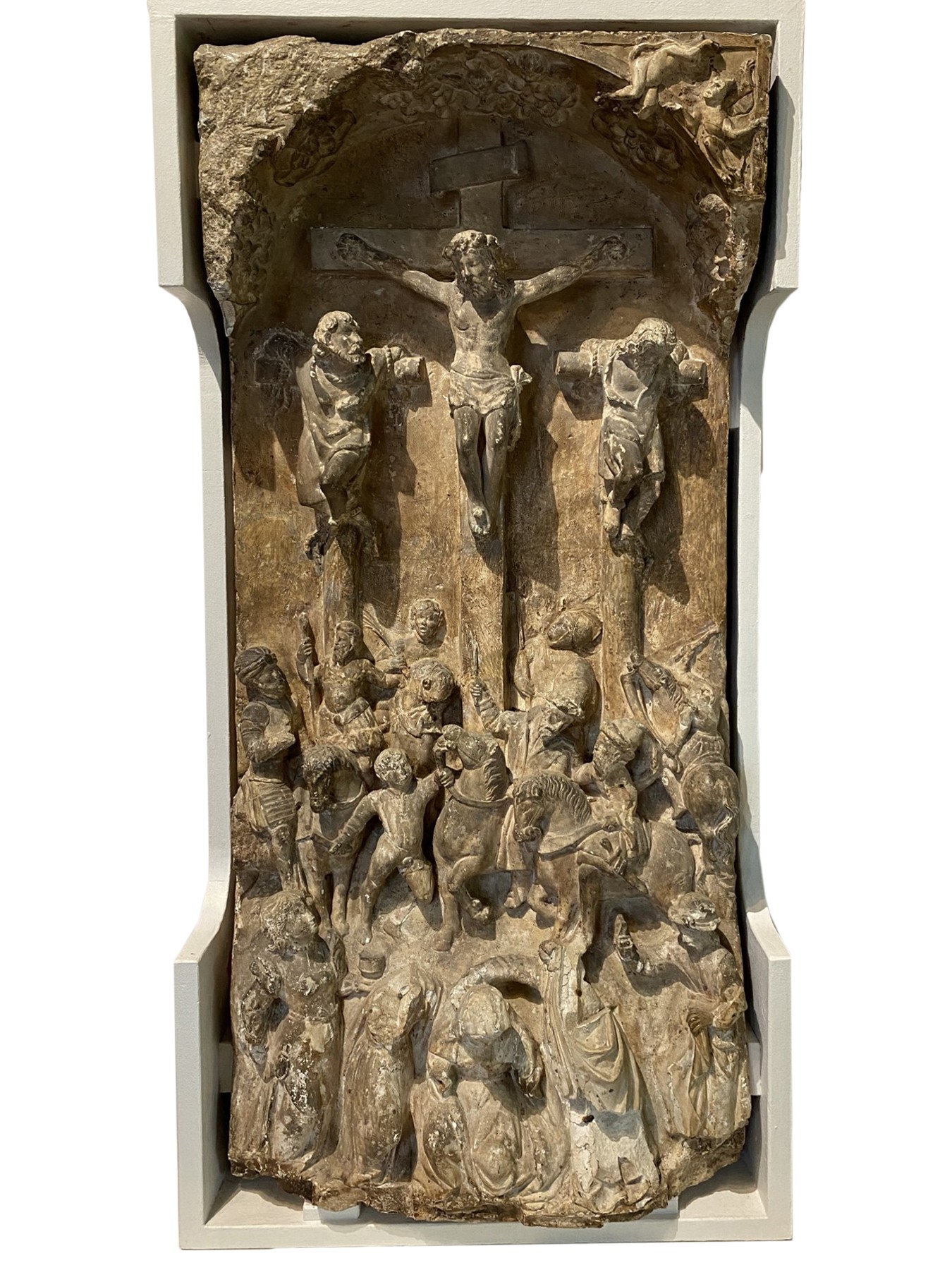This is a color photograph taken outdoors during the day under natural light, presented in portrait orientation. The image captures a 16th-century Renaissance stone relief sculpture, showcasing the Crucifixion of Christ. The carved stone, light brown in color and highly detailed, is encased within a thin-walled wood frame that fits its dimensions perfectly, and the frame itself is concave on both sides. The sculpture features Christ on an ornate central cross with two thieves on either side, one looking up towards Christ. Above the central cross are carvings of angels, though the upper left section has been smoothed out over time. Below the crosses is a multitude of mourners and Roman soldiers, some on horseback. The entire piece is arched at the top, contributing to its intricate and realistic representational style.